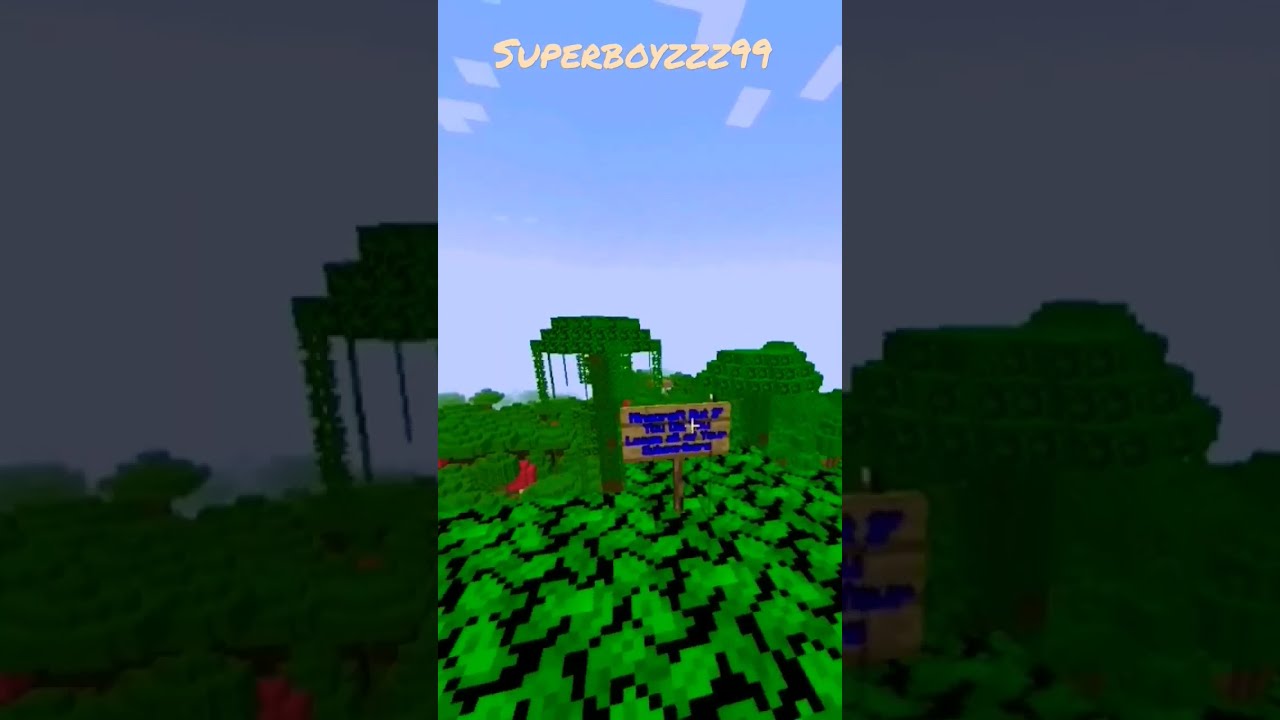This rectangular image appears to be a cartoonish screenshot from a video game, most likely Minecraft, due to its distinct pixelated style and blocky graphics. The view is divided into three sections: left, center, and right. The center section is the primary focus, featuring a clear blue sky with rectangular clouds and the username "SuperboyZZZ99" displayed prominently at the top in a peach or yellow color. Below the sky is a patch of green leaves that seem to form a platform on which several structures are built. 

In the middle of the scene, there's a small brown wooden sign with blue text that is unreadable due to the pixelation and small font size. To the left of the sign, nestled among green foliage, is a red object that could be a tree or potentially a red bird. The background contains various greenish trees, including one particularly tall tree with square-shaped foliage and dangling vines, as well as a wider, pyramid-like tree trunk on the right. The left and right thirds of the image provide close-ups of the tree structures, washed out with dark, semi-transparent colors, contributing to an overall forest-like aesthetic.